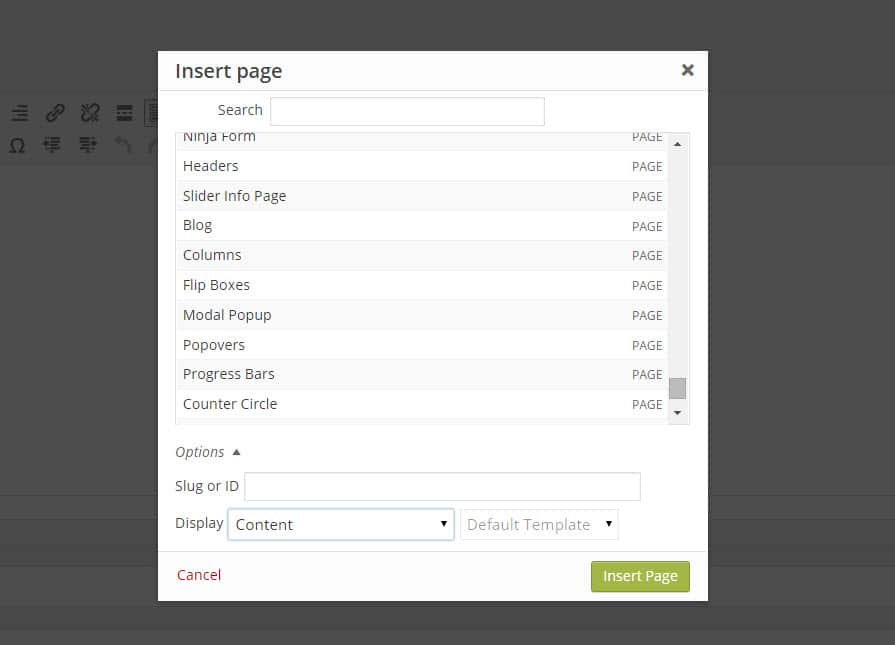A square image showcases a large white box superimposed over a grayed-out desktop area, possibly a Microsoft Word document. The background is heavily desaturated, obscuring most details except for a few discernible icons in the upper left, including a paperclip and a horseshoe-like shape. A prominent white area dominates the center, bordered by grayed-out gray and white bars below it. 

At the top of the white box are the black letters "Insert Page," accompanied by a grayish-black 'X' in the upper right corner. Below this is a faint gray bar followed by the word "Search" next to a long search bar for input. Mid-image, there's a large white area rimmed in faint gray, featuring a vertical scrollbar on the far right. 

This section contains various titles listed in alternating gray and white boxes. From top to bottom, in black text, the titles read:

1. Ninja Form (faintly cut off)
2. Headers
3. Slider Info Page
4. Blog
5. Columns
6. Flip Boxes
7. Model
8. Pop-up
9. Popovers
10. Progress Bars
11. Counter Circle

At the lower left, "Options" is written in italics next to an upward-facing gray triangle. Below that, "Slug or ID" is next to a long white text box. Further down, the word "Display" appears alongside a menu drop-down box labeled "Content," which can be expanded by clicking the downward-facing triangle to its right. Another grayed-out text box next to it reads "Default Template" with a non-interactive black downward-facing triangle.

In the lower section, a faint gray line separates the main area from the footer, where "Cancel" is written in red letters to the lower left, and a green box to the lower right with white letters reads "Insert Page."